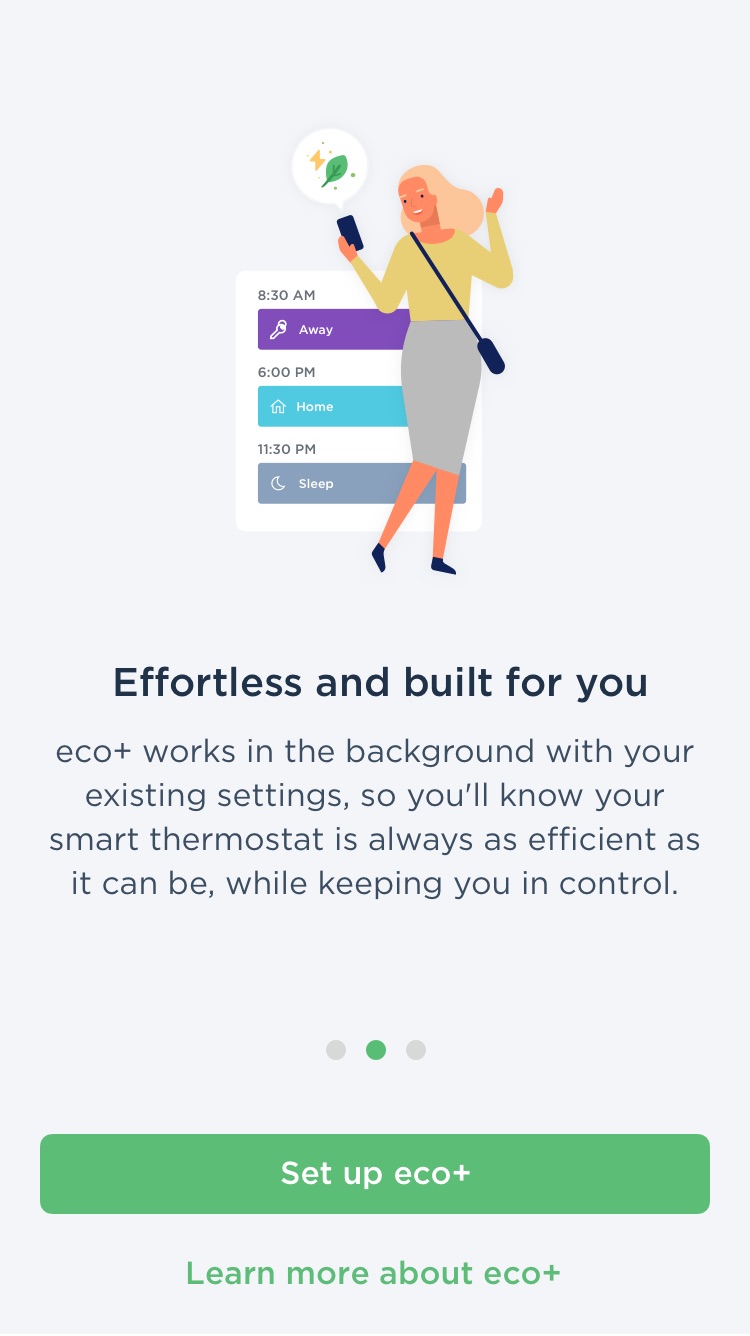This is an advertisement for the EcoPlus app, designed to optimize the efficiency of your existing smart thermostat. The tagline, "Effortless and Built for You," emphasizes its seamless integration and user-centric functionality. EcoPlus operates unobtrusively in the background, ensuring that your thermostat remains as energy-efficient as possible while keeping you in control.

The advertisement features a central illustration of a woman dressed in a stylish skirt and a long-sleeved yellow shirt. She is accessorized with a crossbody purse and is holding a cell phone in one hand, with her other hand raised in a celebratory gesture. Behind her, there is a virtual schedule displayed, showing times and corresponding home statuses: "5:30 AM - Away," "6:00 PM - Home," and "11:30 PM - Sleep."

Below the illustration are three horizontal dots in a row, with the middle dot highlighted in green, signifying an active selection. Beneath this is a prominent green bar containing the call-to-action text "Set Up EcoPlus" in white letters. Further down, in smaller green text, is a link prompting users to "Learn More About EcoPlus." This visually appealing and informative advertisement effectively communicates the app’s benefits and ease of use.